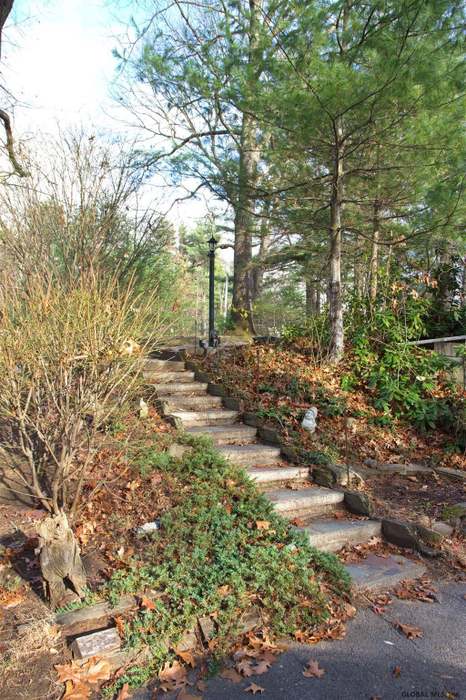The image captures a serene natural scene during the fall season. At the center, a series of cement-gray stairs ascend through a landscape abundant with brown leaves that partially obscure each step. The stairs appear to be around 10 to 15 in number, flanked on both sides by patches of lush green grass dotted with fallen leaves. Bare, brown tree branches frame the scene, hinting at the seasonal transition. In the top left corner, a clear, vivid blue sky is visible, adorned with a few scattered, non-threatening clouds. The bright sunshine bathes the grass, leaves, and trees in a warm glow. On the right side of the image, trees still hold on to some of their leaves, though many are in the process of drifting down, emphasizing the time of year.